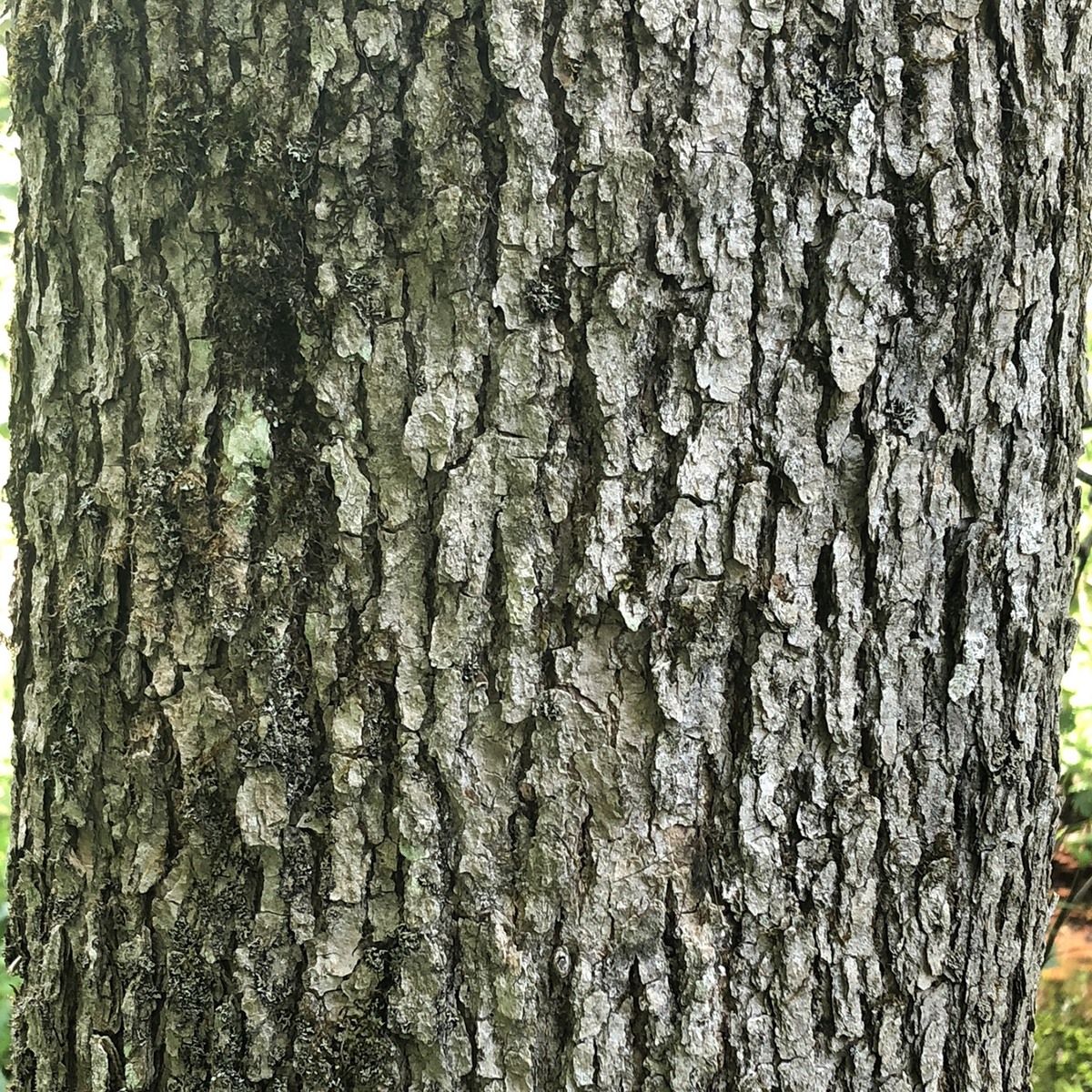The image reveals an extreme close-up of a rough, aged tree trunk, likely from an oak tree. The detailed texture of the bark features numerous cracks, grooves, and pits, giving it an aged, weathered appearance. The bark is predominantly gray with varying shades, including silvery gray, and has moss or possibly some lichen or fungal growths adding subtle greenish hues. These green tints might be influenced by light filtering through the tree's foliage above. Small plants or patches of greenery can be seen peeking from the periphery, but the main focus is the textured surface of the bark. The overall scene exudes a sense of enduring age and natural ruggedness.